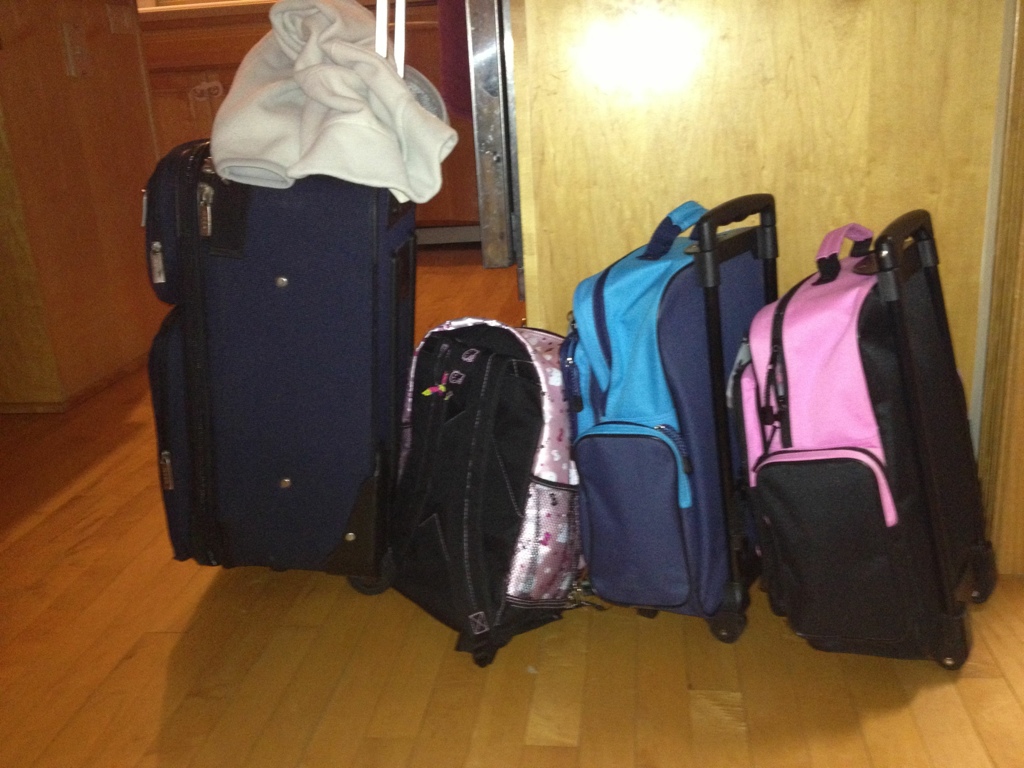In this blurred color snapshot photograph taken in a room with an L-shaped layout, there is a tan wooden floor accompanied by tan light brown painted walls. The background shows a side view of kitchen cabinets, also in a matching tan light brown color. Four pieces of luggage are arranged in a straight line from left to right in the center of the image.

To the far left is a tall navy blue suitcase with wheels and an extended handle, on top of which lies a white long-sleeve shirt or wadded plastic. Next to it, there is a child's shiny satin pink backpack with a black back and white decorations, positioned at a slight diagonal angle. Beside this is a smaller, dark blue and light blue travel backpack with a black collapsed handle and wheels. Far right is another pink and black children's travel backpack with a similar design and features, including a black handle and wheels. The composition is illuminated such that there is a glare or reflection above the luggage from the camera flash, adding to the homely, candid nature of the image.